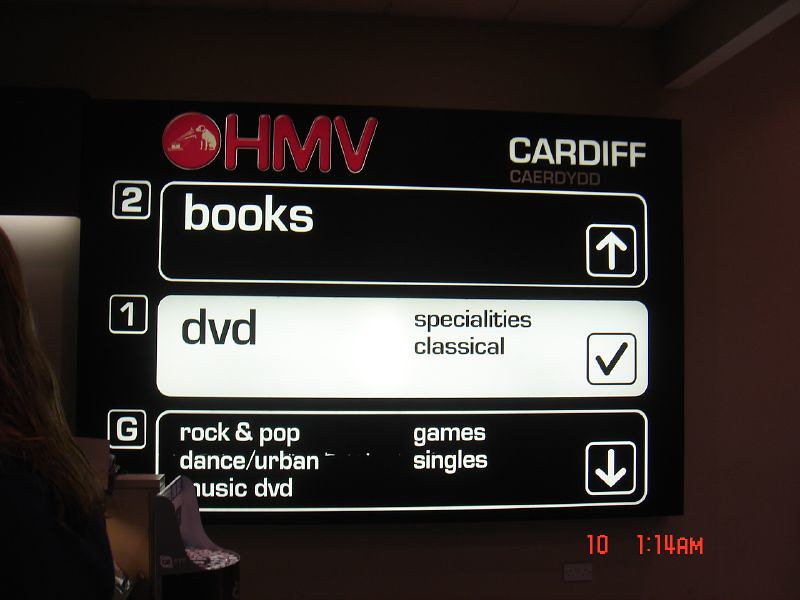The image captures a detailed photograph of an HMV store's directional sign mounted on a dark red wall. The top portion of the sign features the HMV logo in bold red capital letters with a subtle white border, complemented by the name "Cardiff" in white letters to the right, followed by its Welsh equivalent "C-A-E-R-D-Y-D-D" in smaller gray text beneath it. Moving downwards, the sign displays a structured layout for store navigation. A white box with the number "2" indicates the second floor, with the word "Books" and an upward arrow suggesting the location is above. Below, another white box labeled "DVD" features a number "1," signifying specialties and classical sections, alongside a black check mark indicating the current location. Further down, a black box marked with the letter "G" encompasses genres like rock & pop, dance, urban, music DVD, games, and singles, with a downward arrow pointing to these sections. A time stamp reading "10" and "1:14 AM" appears at the bottom. On the left side of the image, the back of a woman's head with long brown hair partially appears, set against the overall store backdrop.